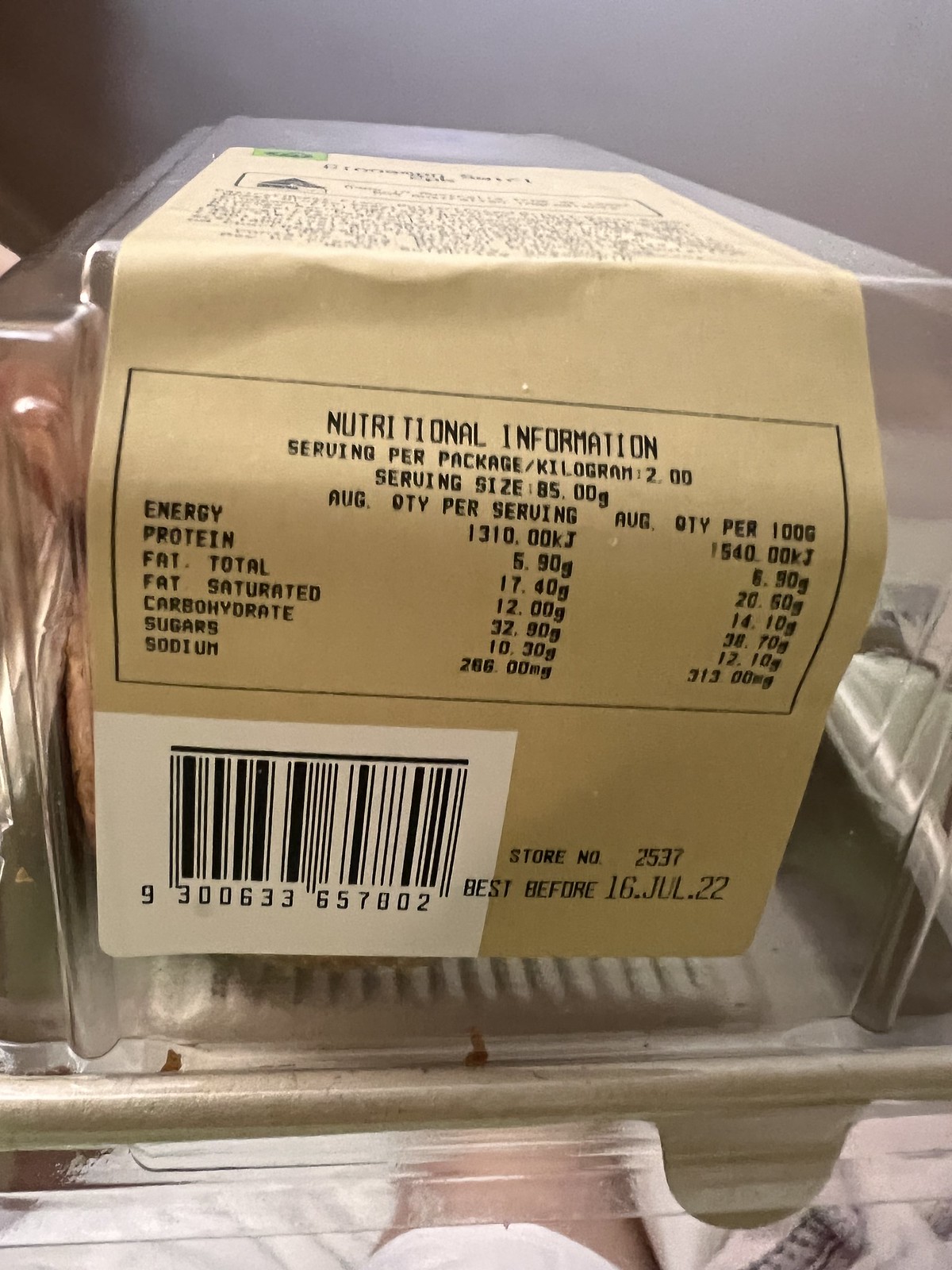This color photograph depicts a clear plastic container with food inside, prominently placed on a shelf. Attached to the container is a cream-colored label with detailed black text. On the left side of the label, a barcode featuring black and white lines is visible, and beside it, the store number 2537 is noted in black letters. The label also displays a “Best Before” date of 16 July 2022.

The central portion of the label is dominated by nutritional information against a light brown background. It specifies servings per package/kilogram as 2, with each serving size being 85 grams. The nutritional breakdown is provided for both average quantity per serving and per 100 grams, listing values for energy, protein, total fat, saturated fat, carbohydrates, sugars, and sodium. The energy content is shown as 1,310 kJ, protein as 5.90 g, total fat as 17.40 g, saturated fat as 12 g, carbohydrates as 32.90 g, sugars as 10.30 g, and sodium as 266 mg, accompanied by their respective per 100 grams values. Above the nutritional details, there's additional text in black lettering that is partially out of view.

The container is situated among many others in a storage setting, with additional containers positioned below and to the sides. The scene provides a comprehensive, detailed view of the product's packaging and labeling, crucial for understanding its nutritional value and expiration information.